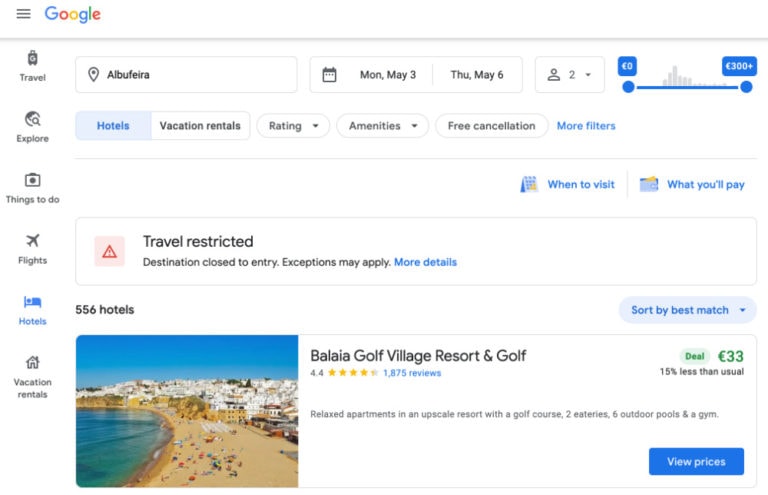The image is a detailed screenshot of a computer screen displaying the results of a Google search for travel accommodations. 

At the top of the screen, there's a three-bar menu icon followed by the Google logo in its characteristic multicolored design. Below this, a horizontal gray line separates the top menu from the content below. 

On the left-hand side, a vertical menu presents various travel-related categories. These include:
1. A suitcase icon labeled "Travel."
2. A globe with a spyglass icon labeled "Explore."
3. A list item labeled "Things to Do."
4. An airplane icon labeled "Flights."
5. An icon of a bed with a person in it, labeled "Hotels."
6. An icon of a house labeled "Vacation Rentals."

At the top of the main section, there are several input and filter options. This screenshot shows a search for "alberia," with travel dates from May 3rd to May 6th, specifying the number of people and a price range. Below these inputs, several filter buttons are visible, including "Hotels," "Vacation Rentals," and dropdown menus for "Rating" and "Amenities." There is also a notable blue text link labeled "More filters."

Another gray dividing line separates the input section from additional information below. This includes a "When to Visit" calendar, a section on "What You'll Pay," and a highlighted advisory box. The advisory box features an exclamation mark inside a triangle with the text "Travel restricted. Destination closed to entry. Exceptions may apply," followed by a clickable "More details" link for further information.

Finally, the search results show a total of 556 hotels, sorted by "Best Match" through a dropdown menu. An example result shows a picture of a resort, the name of the resort, the deal price, and a call-to-action button labeled "View Prices."